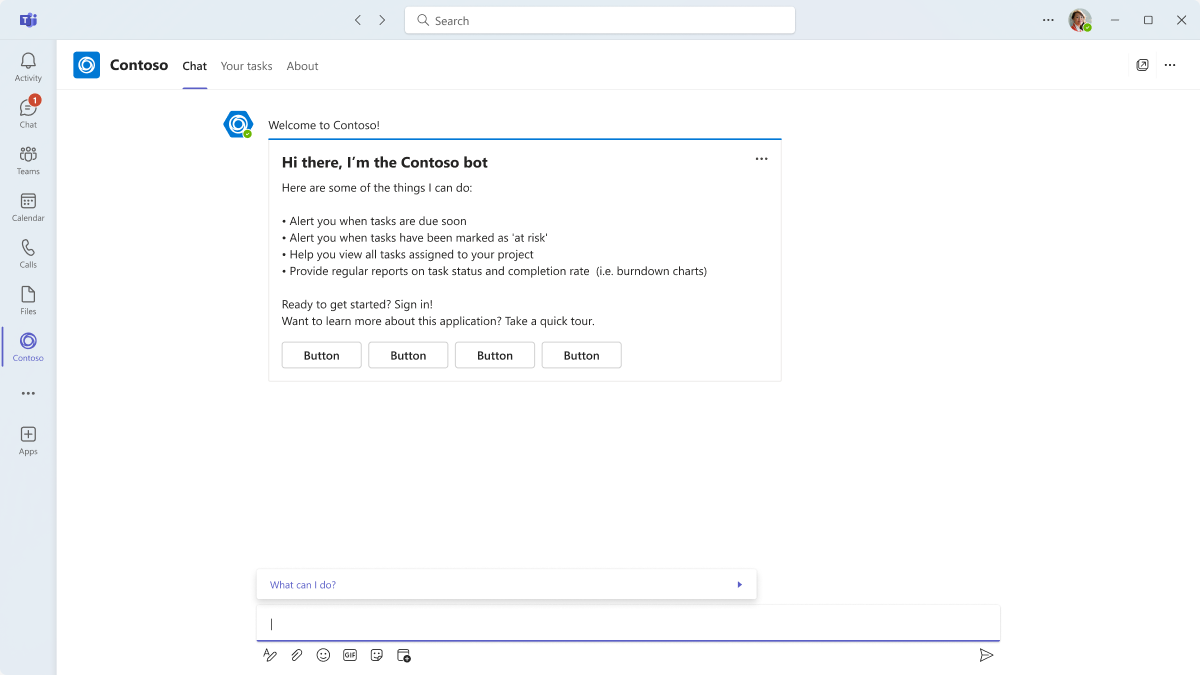This is an image showing a page from the Contoso website. On the left side of the page is the Contoso logo, which consists of a blue square enclosing a white circle with blue lines inside it. Along the left border, there’s a vertical tab column featuring several icons: a notification bell, a chat bell with the number one indicating an unread message, the Microsoft Teams logo, a calendar icon, a calls icon, a files icon, and another Contoso logo. Below these icons are three vertical dots followed by three horizontal dots, a plus sign labeled "Apps," and additional navigation options.

The main content of the page is divided into four tabs situated at the top: "Chat," "Your Tasks," "About," and an unnamed tab, with the "Chat" tab currently active. On the right side of this main section, there are three horizontal dots and a pop-up window. The pop-up reads: "Welcome to Contoso!" followed by a blue dividing line and the text: "Hi there, I'm the Contoso bot." It continues with a list of services the Contoso bot can provide. These services include: alerting users when tasks are due soon, alerting users when tasks have been marked as high-risk, helping users view all tasks assigned to their project, and providing regular reports on task status and completion rates, such as burn-down charts.

At the bottom of the pop-up, there are prompts to "Sign in" to get started and a call to "Take a quick tour" for more information about the application. There are also four placeholder buttons simply labeled "button." Finally, below this section, there’s an input box with the label "What can I do?" suggesting an area where users can type in questions or commands, indicated by a blinking text cursor.